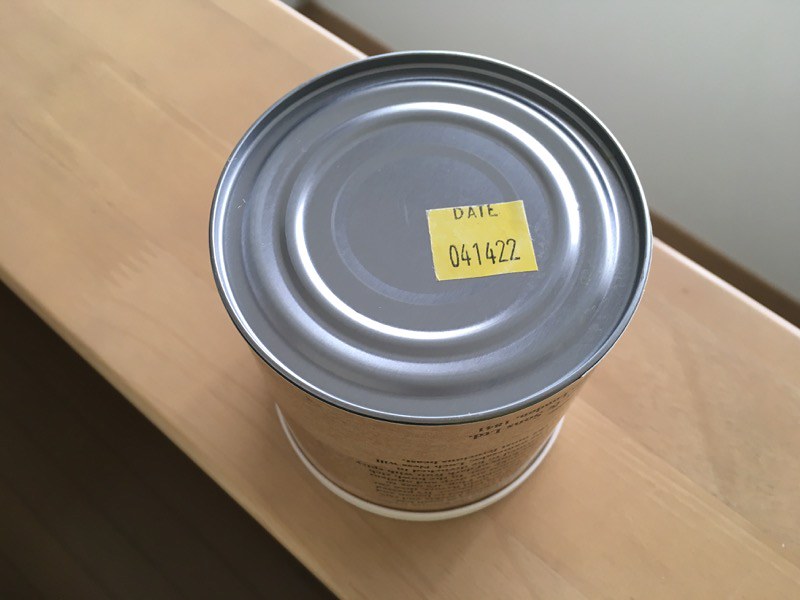An overhead view shows an unopened can positioned on a light tan board. The can features a silver, slightly reflective top adorned with a rectangular yellow sticker that reads "date 041422" in black lettering. The can's label is tan with black writing, though the overhead perspective obscures the specifics of the text. Adjacent to the board is a gray surface, possibly part of a table. Below the board lies a dark surface composed of narrow strips, adding contrast to the scene.